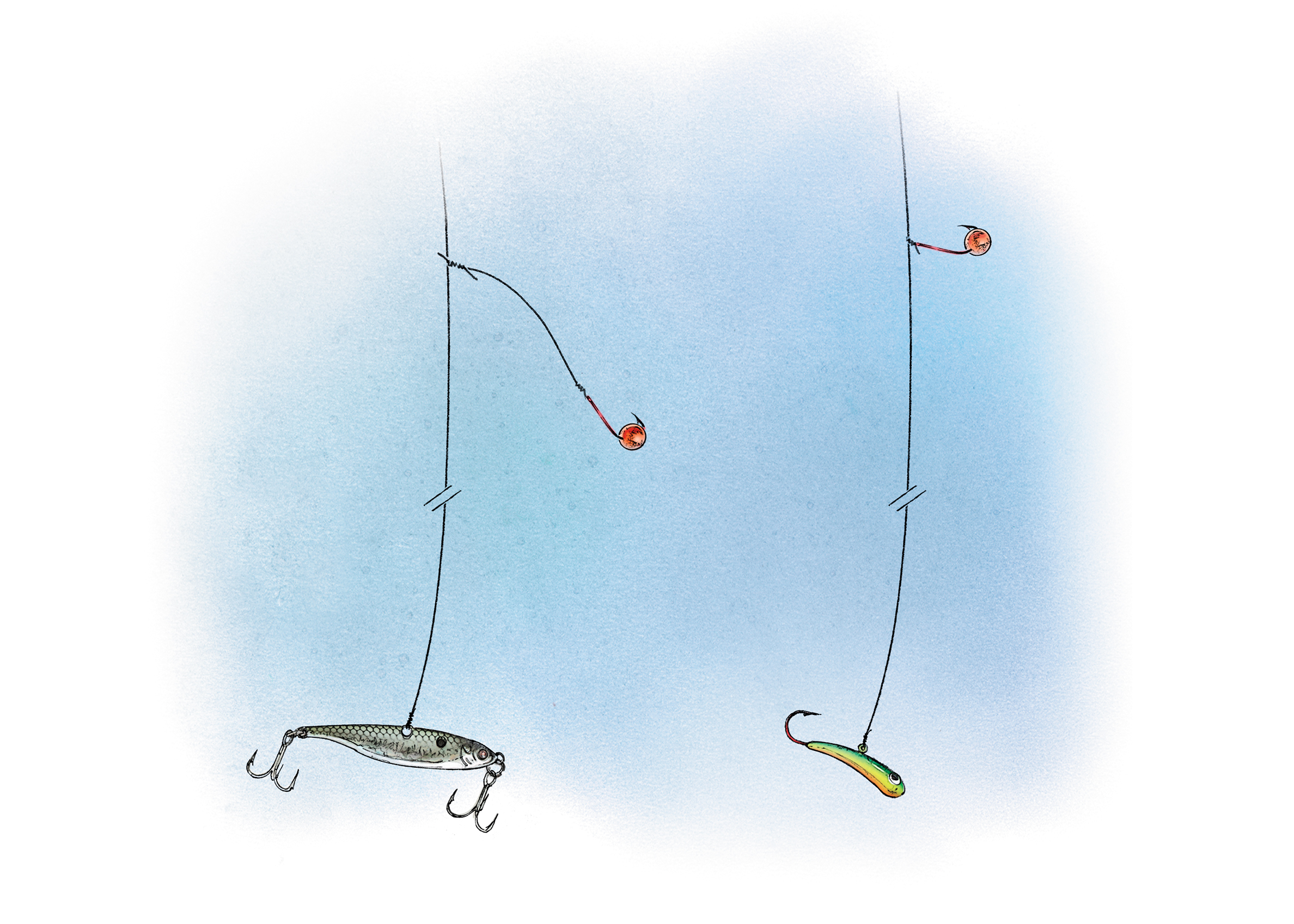This illustration depicts two fishing lures against a light blue, watercolor-like background with an irregular, hazy circular shape. Both fishing lines descend from the top of the image, each showcasing unique lures and hooks. The left line features a lure shaped like a silvery fish, resembling a sardine, with detailed markings including an eye and a tail. Two identical metal hooks emerge from both its nose and tail. The hooks have a triangular base with three curved prongs each. Midway up, the fishing line is interrupted by a broken section, suggesting additional length not shown in the image. Extending from this part, a separate string moves to the right, ending in a small red ball with a metal prong.

The right fishing line is similar in structure but hosts a differently styled, multicolored lure. This hook, vibrant with shades of green, yellow, and orange, resembles a cartoonish fish with an eye mark. It features a single curved hook extending from its tail. Like the left line, the right line also includes a break mid-length, and from this break, another shorter string angles rightward, also ending in a red ball and prong setup. Both lures' distinctive designs and the various hooks paint a detailed and vivid image of the fishing equipment.